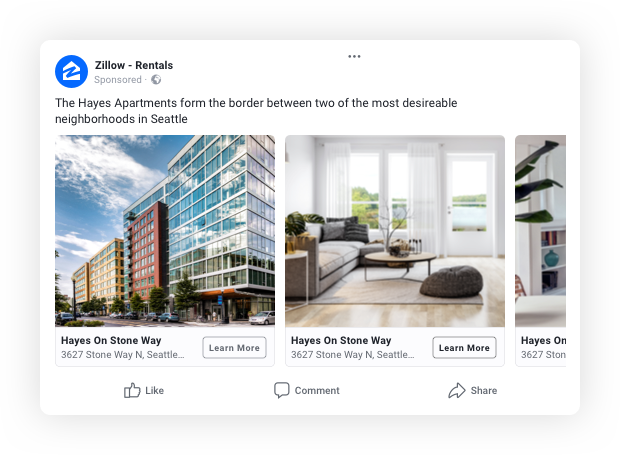The image depicts a computer screen displaying the Zillow Rentals website, characterized by a white background. At the top center of the screen, three gray dots can be seen. Beneath these dots, on the far left, a medium blue circle contains a white house icon with a blue 'Z' superimposed over it. To the right of this icon, in dark type, it reads "Zillow - Rentals." Below this, it says "Sponsored" in light gray text, followed by a gray world icon.

In dark type, a description below this icon reads: "The Hayes Apartments form the border between two of the most desirable neighborhoods in Seattle." 

The main part of the screen is divided into two large panes with a third one partially visible on the right. The left pane displays a city scene with a bright blue sky and clouds, showcasing several multi-story buildings. The buildings vary in color and style: a yellow one in the distance, a red one in the center, and a prominently featured glass building on the right that appears to be eight or nine stories tall. Below this image, it is labeled in dark type as "Hayes on Stoneway." Beneath this label, it further specifies in light gray text: "3627 Stoneway North, Seattle." There’s also a clickable gray box outlined in gray with the text "Learn More" in the center.

The right pane shows an interior view of the same apartment. Identified at the bottom with the same labels, "Hayes on Stoneway" and "3627 Stoneway North, Seattle," it also includes a "Learn More" box. The image reveals a cozy living room with a couch to the left adorned with cushions, large windows with white curtains straight ahead, and a door leading outside, where greenery is visible. The room features a rug, a table, a chair, and light wood flooring.

To the far right, partially cut off, another photograph of the same property is visible, showing a bit of the interior with a white wall, white bookcases filled with items, and a plant.

At the bottom of the screen, there are three interactive icons: a thumbs-up icon labeled "Like" on the left, a comment bubble icon labeled "Comment" in the center, and a rightward arrow icon labeled "Share" on the right.